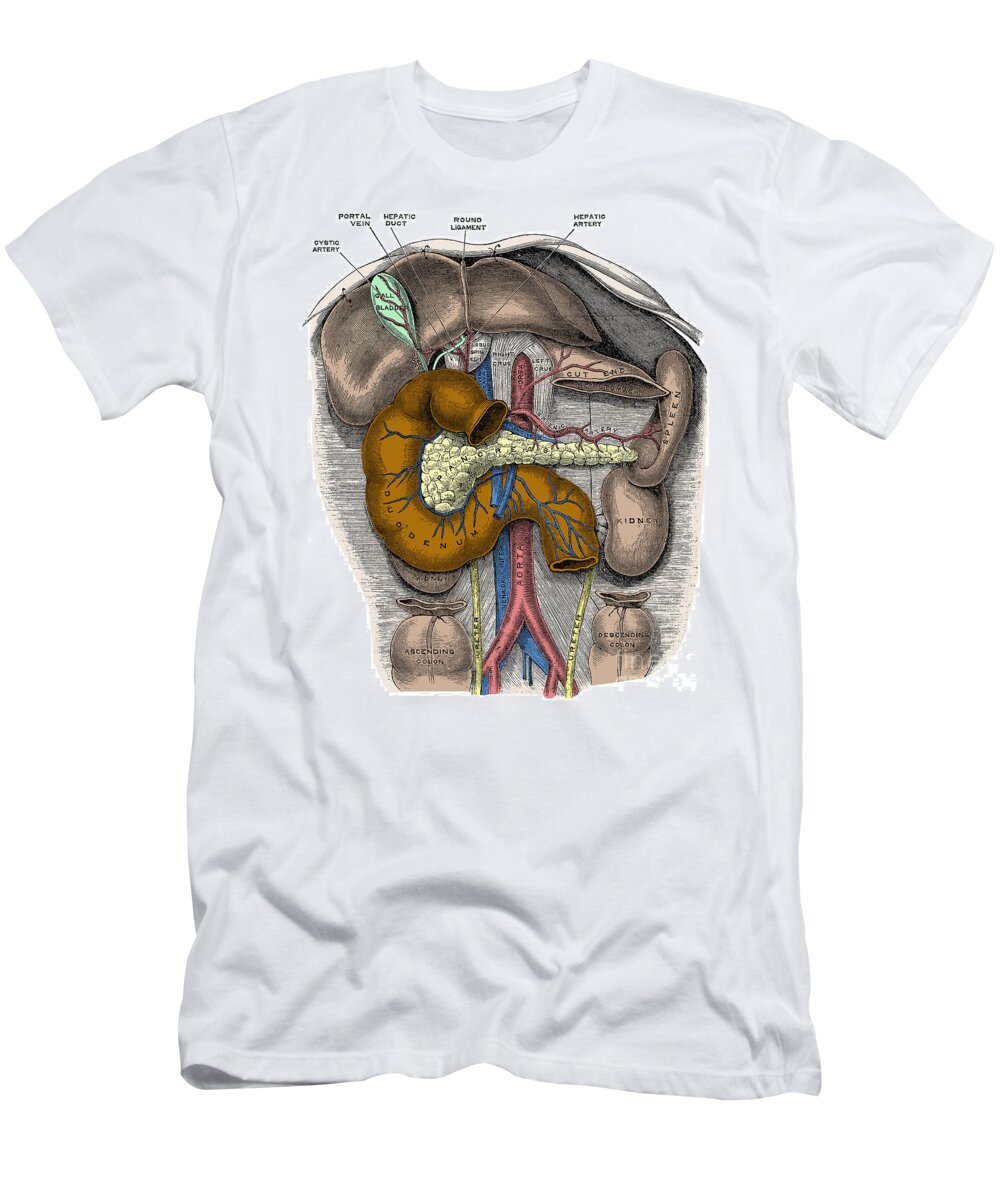This image depicts a white, short-sleeved t-shirt with a detailed illustration of the human body's internal organs printed on it. The t-shirt design, set against a perfectly white background, spans from the chest area down to around the belly button, capturing a significant portion of the upper torso. Various anatomical structures are meticulously labeled in the diagram, including the cystic artery, portal vein, hepatic duct, round ligament, hepatic artery, gallbladder (highlighted in a mint green color), spleen, kidneys, and sections of both the ascending and descending colon. The pancreas is indicated in white, while the duodenum is shown in a mustard yellow-brown hue. Blues and reds trace the pathways of arteries and veins throughout the image. The background of the illustration features subtle horizontal lines, adding texture to the overall design. The shirt itself displays some natural wrinkles at the bottom, creating realistic lighting and shadow effects. The scientific accuracy and the array of organ depictions make this t-shirt a unique representation of the human digestive system and related anatomy.